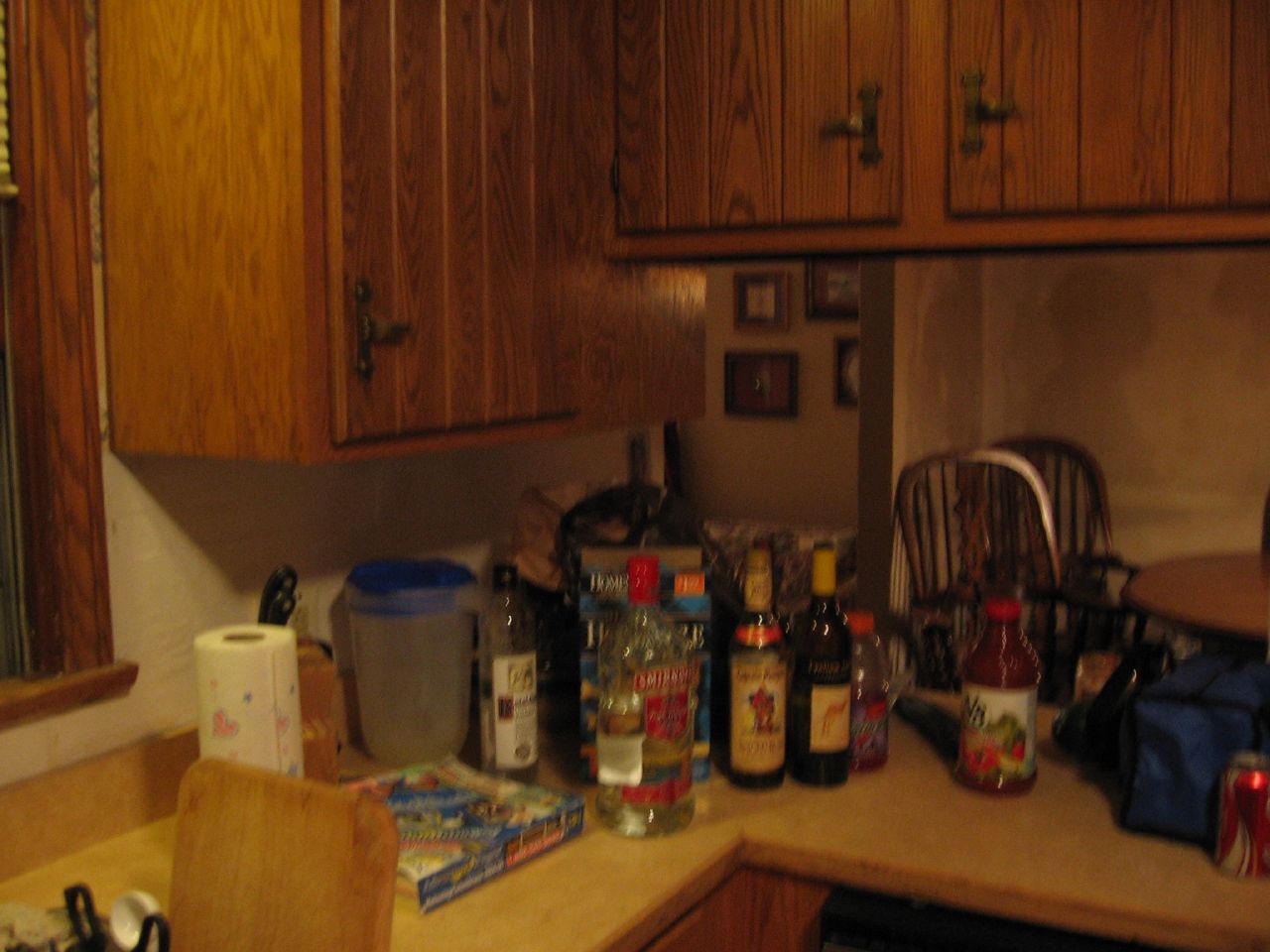The image depicts a slightly blurry, evening scene of a kitchen corner, with dimensions suggesting it is wider than it is tall by approximately 20%. At about 60% from the left, the countertop makes a corner. The countertop itself is light brown, accompanied by medium brown cabinetry both below and overhead. To the left, a window with medium brown trim is present, indicating it is night outside due to the visible darkness.

The countertop hosts various items. Prominently, there are several alcohol bottles, including recognizable brands like Captain Morgan and Smirnoff, among others that are indistinct. There are about five bottles in total. On the left side, a semi-clear container with a blue lid is visible next to a roll of paper towels. A bottle of V8 juice sits on the right side. In front of the container on the left side, a board game is discernible. 

Above the counter on the right-hand side, four small pictures are neatly hung on the wall just beneath the overhead cabinet. Towards the right edge of the frame, a portion of a blue duffel bag is visible, mostly cut off by the image’s border. In front of the duffel bag, a can of Coke is partially cut off by the image’s edge.